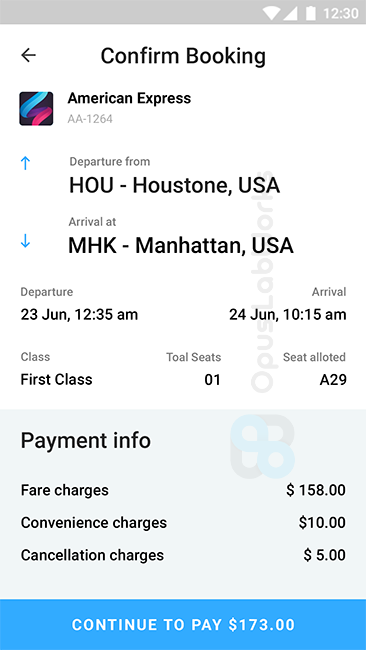In this image, we see a screenshot taken on a smartphone, displaying the details of an air flight booking. The top right corner shows the current time as 12:30, with a fully charged battery icon at 100%, a fully strong cell signal, and a fully strong Wi-Fi signal. 

Centered at the top of the image is the text "Confirm Booking," with a left-pointing arrow to its immediate left. Below this, it reads "American Express AA-1264," and to the left of this text is a small squared box featuring a wavy design in blue, purple, and pink colors.

Further down, the text specifies the flight's departure from "Houston-Houston USA" and its arrival at "MHK-Manhattan USA." In the middle section of the image, the departure time is noted as "23 June 12:35 AM," and the arrival time as "24 June 10:15 AM."

At the very bottom of the screenshot, there's a blue box containing the prompt "Continue to Pay $173" in white text.